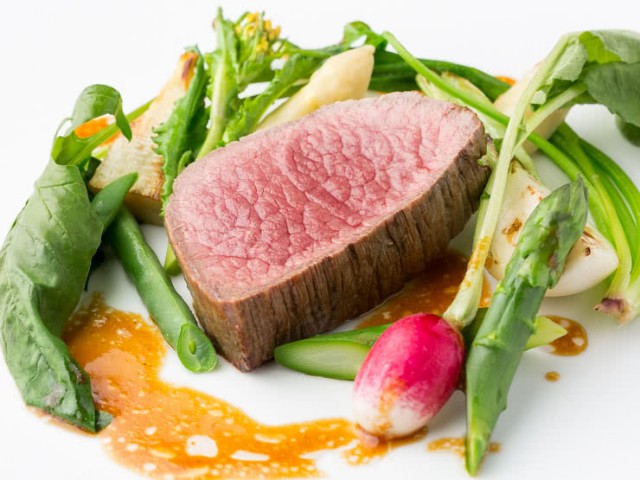This close-up photograph showcases a gourmet dish with meticulous presentation, likely from a Michelin-star-level restaurant. At the center is an almost triangular slice of beef fillet, seasoned to medium with a brown exterior and a light pink interior, approximately an inch thick. The beef is garnished with delicate green leaves and surrounded by an array of vegetables, including pink and white turnip, small red radish, and asparagus tips. A drizzle of brown and orange sauce elegantly accents the plate, adding a contrast of color to the pristine white background. The overall minimalistic and avant-garde design highlights both the quality of the ingredients and the sophistication of the culinary craftsmanship.